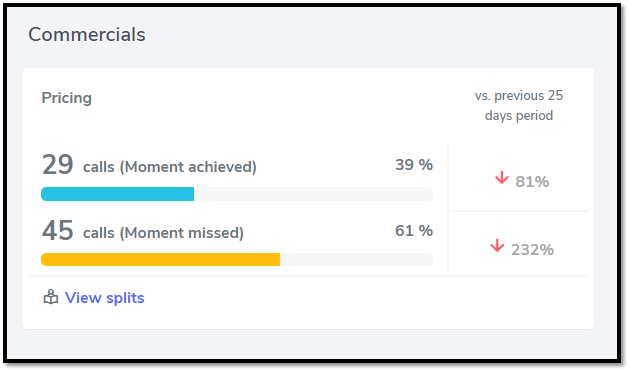An image of a blackboard is filled with various commercial metrics and graphical elements. At the very top left corner, labeled "Commercials," you can see a comparison of pricing versus the previous 25-day period. 

Here are the detailed numbers and their respective visual representations:
- 29 calls are listed, each marked as "moment cheat," illustrated by a blue bar filled to 39%.
- Next to this, an arrow points downward, labeled 81%, with 45 calls marked as "moment missed," accompanied by a yellow bar filled completely to indicate 61%.
- Another downward arrow shows a significant rise to 232%.

The display also includes a section labeled "View Splits," marked with a white square in the background. The edges of the blackboard are fully adorned with lines and textual data, maintaining a neat layout around the metrics.